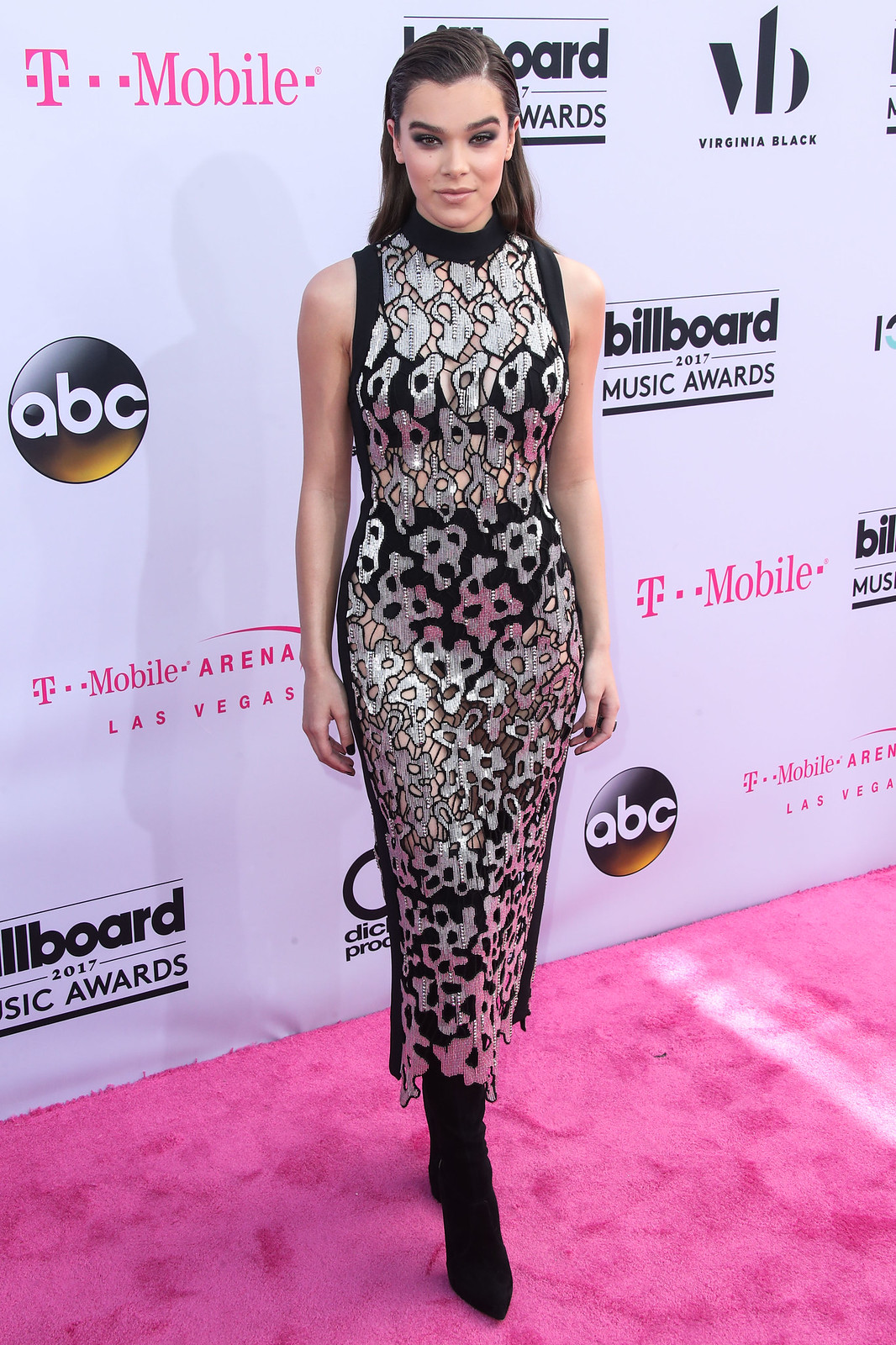This image captures actress Hailee Steinfeld at the Billboard Music Awards 2017 in Las Vegas, standing on a bright pink carpet sponsored by T-Mobile. She is dressed in a sleeveless, slender silver and black dress adorned with intricate designs and shapes, which reaches down to her ankles. Complementing her dress, she wears long, black, velvety boots. Hailee's dark hair is combed back, enhancing her overall elegant look, and her makeup adds to her charm. She stands confidently, her hands resting by her side and offering a subtle, close-lipped smile. The backdrop behind her is a white wall densely populated with various advertisements including the ABC logo, T-Mobile, "Arena Las Vegas," "Billboard Music Awards 2017," and Virginia Black (VB).